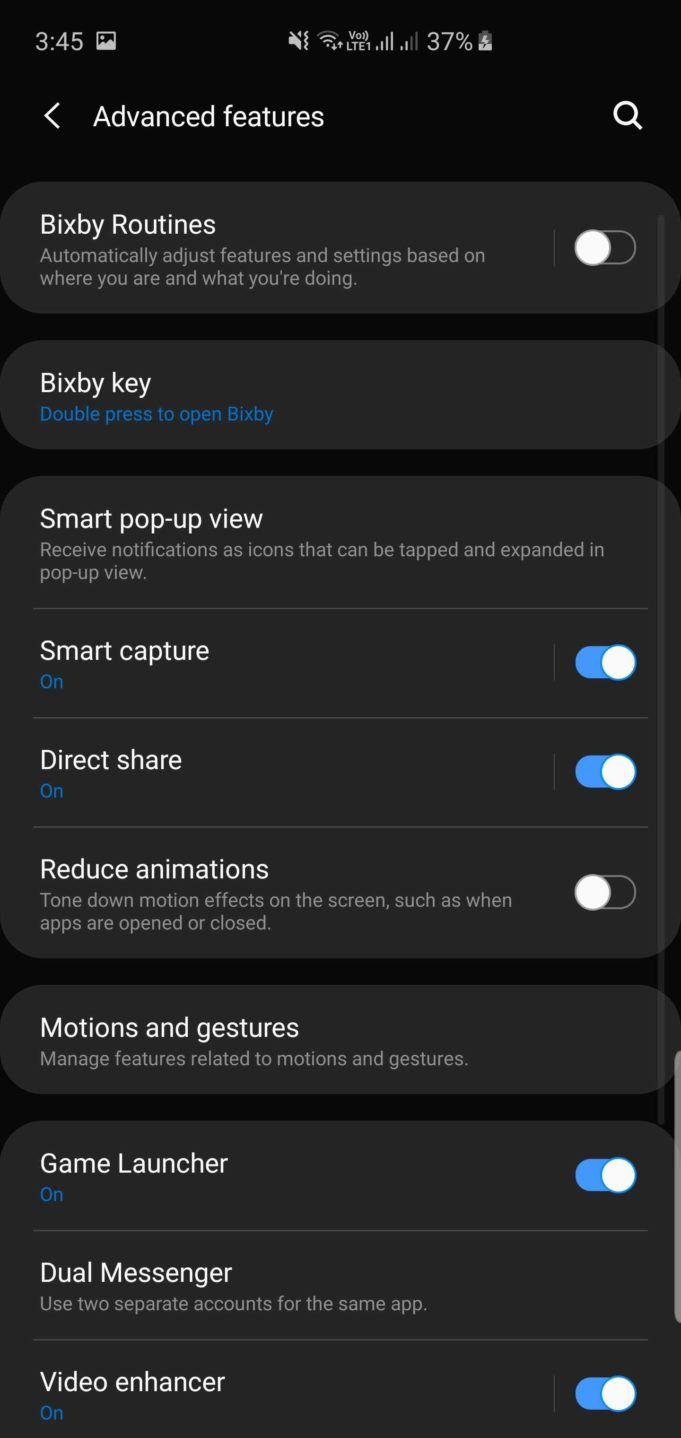This is a detailed screenshot of a smartphone's "Advanced Features" settings page, displayed in dark mode with a black background. At the top left corner, an arrow icon and the "Advanced Features" text are visible, indicating a navigational option. To the right, there is a search icon for easy access to settings.

Directly below, there are several settings options organized with toggle switches. Each setting is labeled with white text within dark gray ovals:

- **Bixby Routines:** This option is turned off.
- **Bixby Key:** This is set to double-press in order to open Bixby.
- **Smart Pop-Up View**
- **Smart Capture:** This is turned on.
- **Direct Share:** This is turned on.
- **Reduce Animations:** This is turned off.
- **Motions and Gestures**
- **Game Launcher:** This is turned on.
- **Dual Messenger**
- **Video Enhancer:** This is turned on.

In the upper left corner of the screen, the time is displayed as 3:45. On the upper right corner, the battery level is shown to be at 37%.